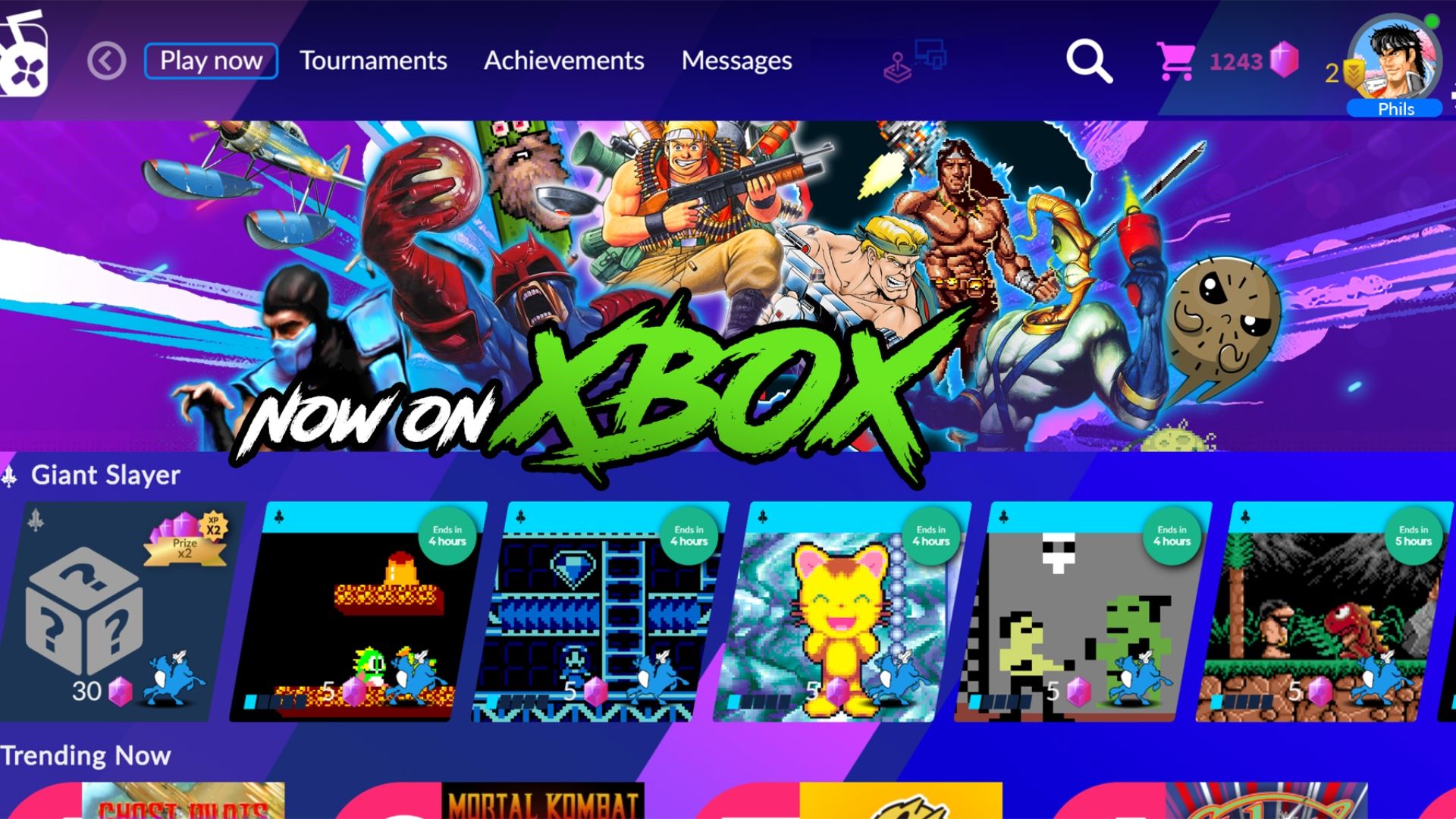This image appears to be a vibrant and detailed menu screen for Xbox, possibly from a streaming service akin to Netflix for video games. The prominent feature is a large colorful banner with a purple background showcasing a collage of various iconic video game characters. Notably, the characters include Sub-Zero from Mortal Kombat, Earthworm Jim in his muscular spacesuit, a commando-like figure with a cigar and blonde hair possibly from Metal Slug, and a character resembling a daredevil. There are also cartoonish and pixelated characters such as a pickle-like entity with a beard, a barbarian, a brown meatball-like creature, and a character in a blue spandex suit holding a ball. 

The upper left of the screen displays selectable options such as "Play Now," "Tournaments," "Achievements," and "Messages." In graffiti-style white text, it reads "Now on" followed by "Xbox" in green text. Below the character collage, banners advertise trending games like "Giant Slayer" alongside an assortment of game selections, including what seem to be 8-bit titles evocative of classic Nintendo games. The overall color scheme is dominated by blues and greens, giving it a lively and engaging appearance. This screenshot encapsulates the dynamic interface and diverse game offerings of the Xbox platform.